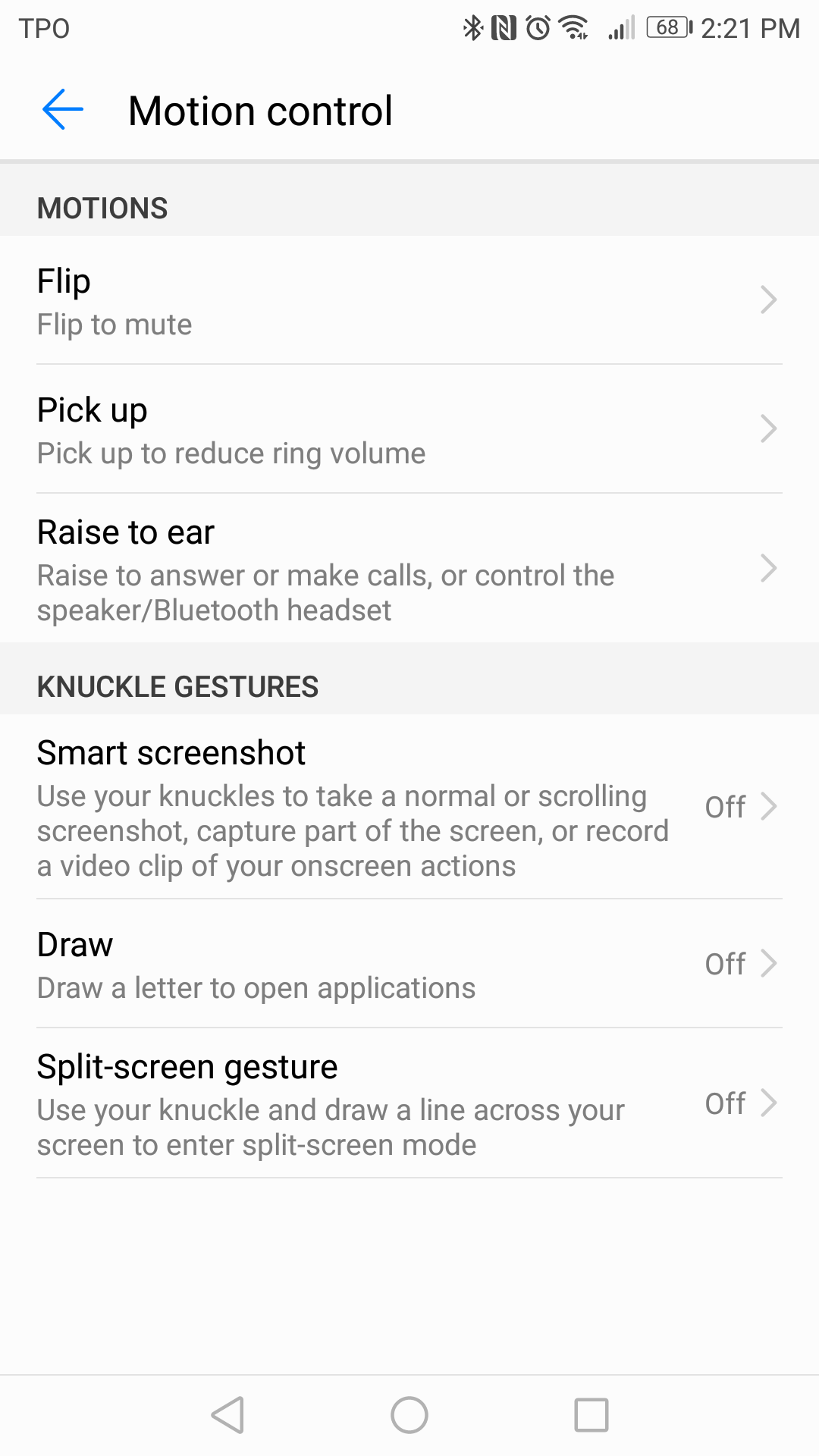The screenshot captures the interface of a mobile phone at 2:21 PM, as indicated by the clock icon at the top right corner. The battery icon beside it shows a 68% charge. Following to the left, the status bar features several icons: a signal strength icon with 3 out of 5 bars, a fully filled Wi-Fi icon, an alarm clock icon, and a Bluetooth icon.

On the top left, the mobile carrier is indicated with "TPO." Below this, a blue arrow points left next to the words "Motion Control." The screen is divided into several sections, with "Motions" as the first main category. Under "Motions," three subcategories are listed: "Flip," "Pick Up," and "Raise to Ear." The next main category is "Knuckle Gestures," which includes subcategories such as "Smart Screenshot," "Draw," and "Split Screen Gesture."

At the bottom of the screenshot, there are three navigation icons: a left-pointing arrow, a circle, and a square, which are likely for back, home, and recent apps functions respectively.